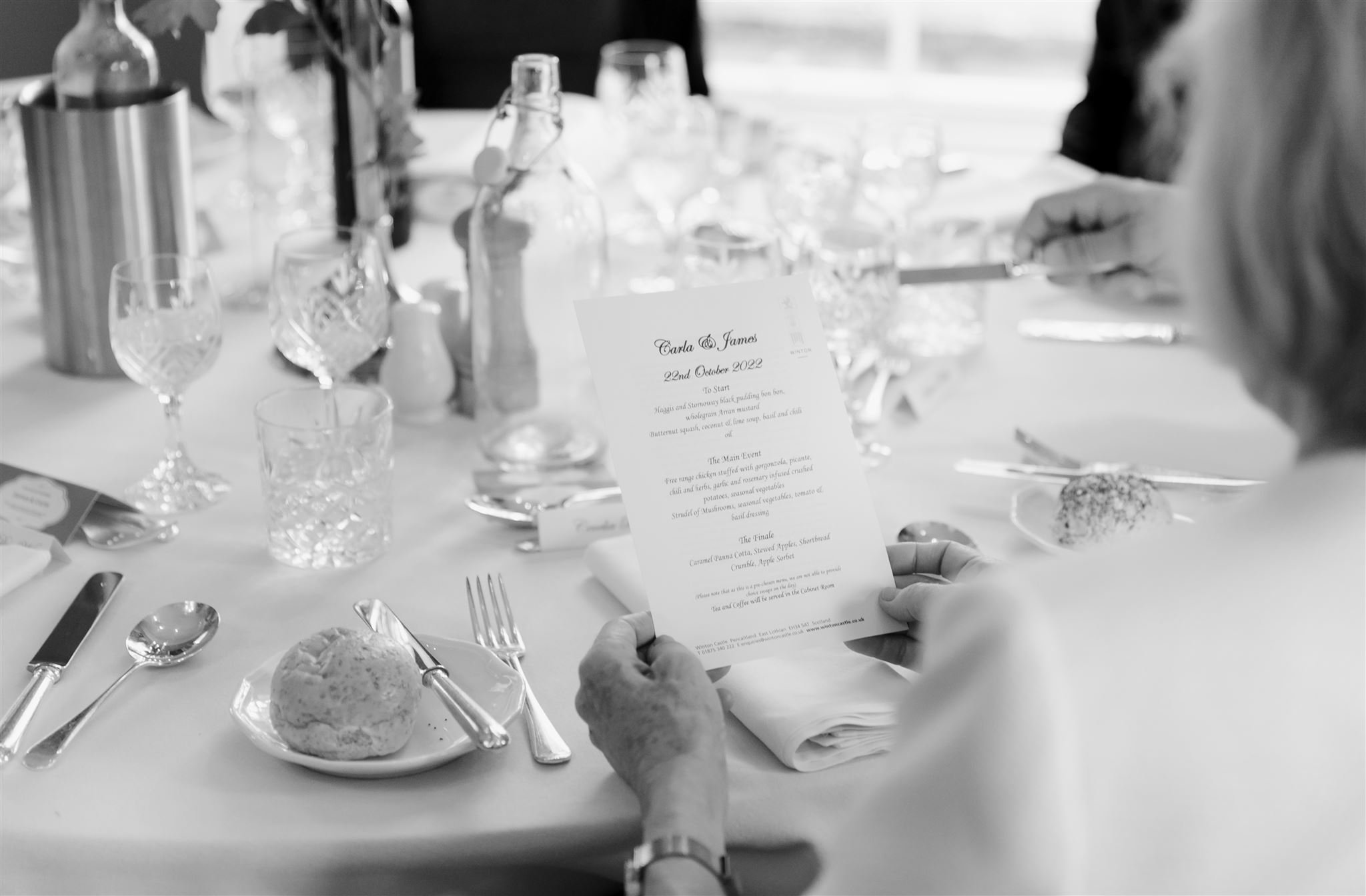The black-and-white photograph captures an elegant indoor setting, likely a high-end restaurant or cafe, seen from the perspective over a woman’s shoulder. The woman is holding a rectangular menu or invitation that reads "Carla A. James, 22nd October 2022." The menu details are partially visible, listing "To start, haggis and strawberry black pudding," "the main event, free-range chicken," and "the finale, caramel pan kata," though much remains too low-res to decipher. The spacious round table, draped in a white tablecloth, is meticulously set with an array of cutlery, wine glasses, and other glassware. Visible are also glass bottles, a nearly empty wine bottle, and small plates with bread rolls and butter knives. The setting suggests a formal meal, perhaps a celebration or wedding, with multiple place settings indicating a gathering of numerous guests. In the background, additional diners can be glimpsed, emphasizing the communal and festive atmosphere of the occasion.